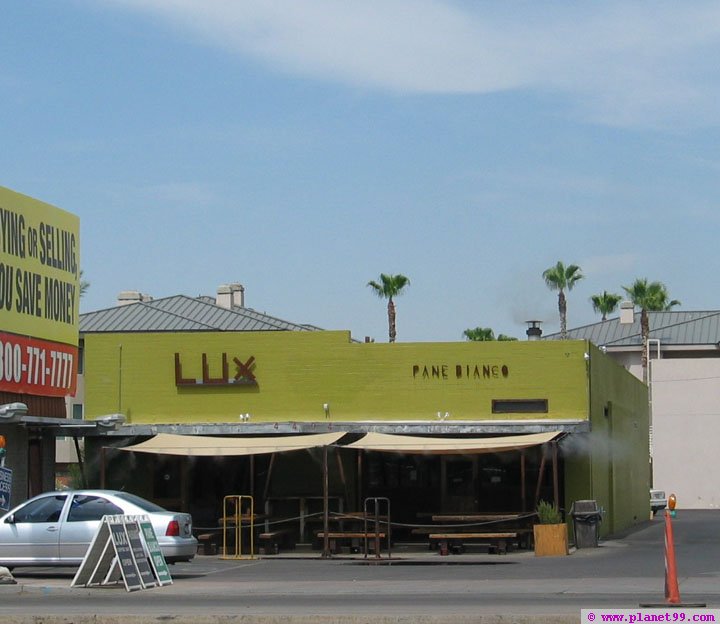The image shows a storefront or a building painted in a vibrant mustard yellow color. Prominently displayed on the left side of the building is a bold, angular red sign that reads "LUX," with the "L" and "U" in uppercase and the "X" smaller and blockier. To the right side, there is a subtler sign for "Pane Bianco" in a different font and smaller text size. The building features a couple of canvas awnings extending from the front, providing shade over several picnic tables and a planter. In front of the building is a silver 90s sedan parked next to a trash can.

The scene is framed by a mostly clear, lightly hazy blue sky, which occupies around 60% of the image. A few thin clouds dot the sky, while palm trees stand out against the backdrop of white buildings with gray roofs behind the main building. To the far left, part of a yellow and red billboard is visible, with the words "selling" and "save money" discernible, along with a phone number in red lettering.

Additionally, there are several advertising placards near the storefront, two of which are white with black images, and one is green. These placards appear to be related to the LUX storefront.